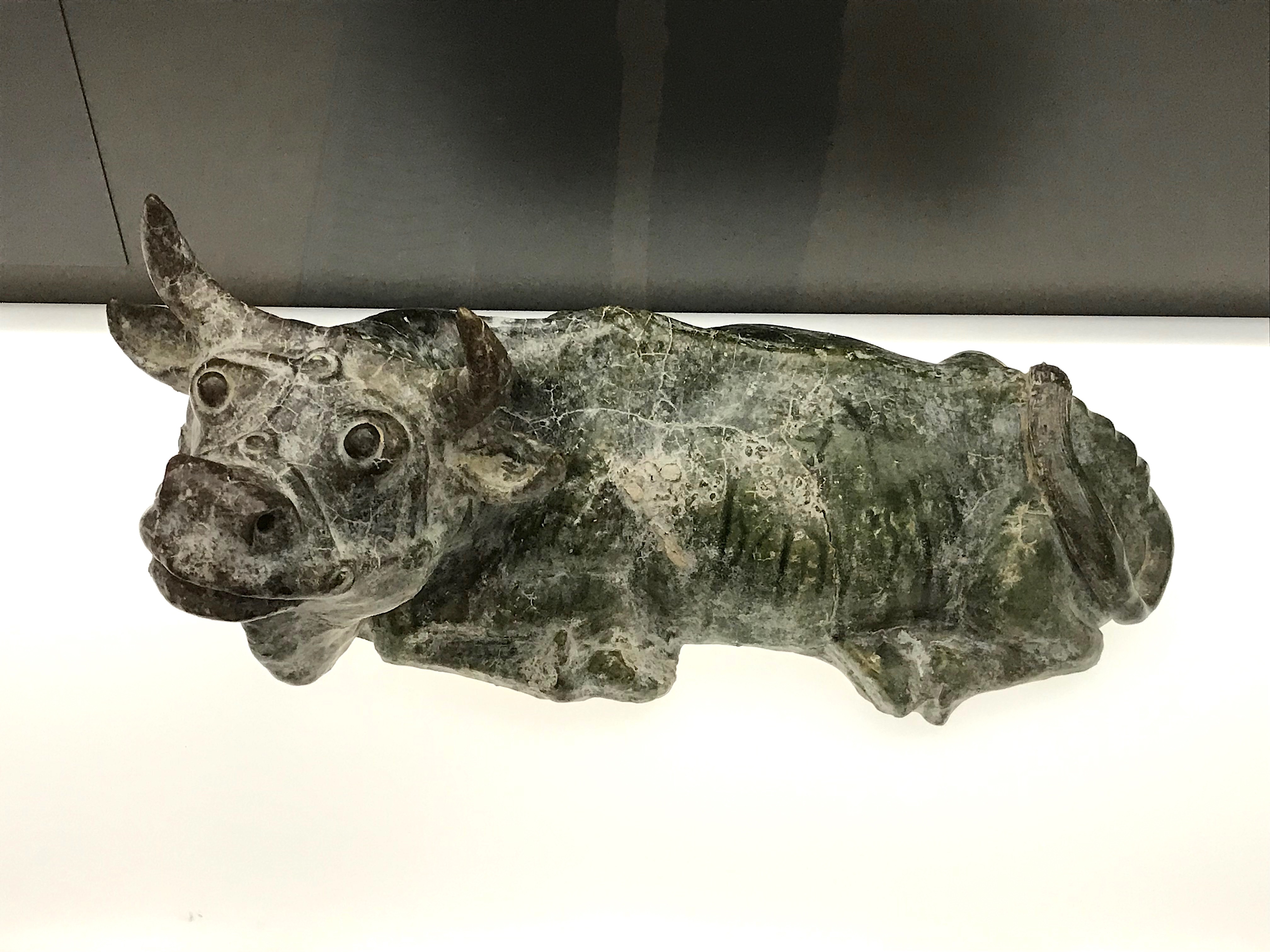The image features an ancient-looking ceramic figure of a reclining bull, centrally placed on a reflective white platform. The bull’s body showcases a combination of faded green, dark brown, and gray hues, with noticeable white scratches or lines that suggest age and wear. The bull’s detailed features include two intact horns, large curved ears, expressive eyes, noticeable nostrils, and a mouth. Its legs are tucked beneath it, and a tail is visible extending to one side. The figure is oriented to the left, giving it a contemplative and somewhat cute appearance. The backdrop consists of a black and brown wall that appears to be a piece of black cloth with varying textures. Despite its detailed depiction, the bull casts no shadow on the platform, enhancing the focus on the figure itself.